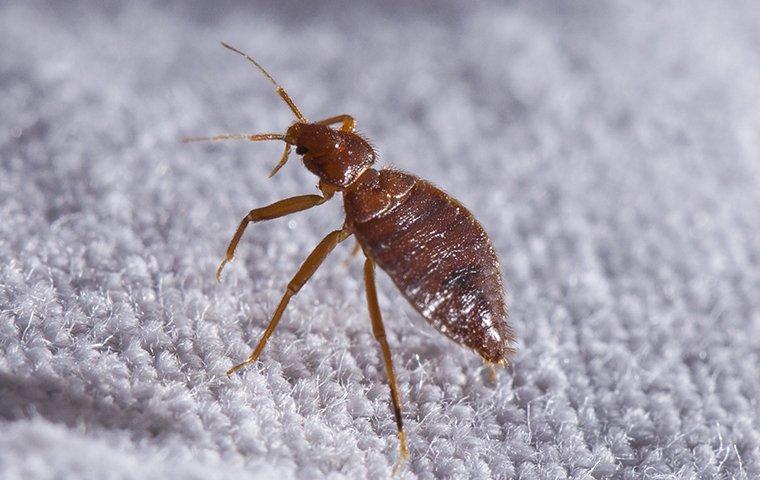This is a zoomed-in and detailed photo of a brown, leaf-shaped bed bug with a small head and two long antennae protruding from its nose. The insect has six skinny legs, with what appears to be spikes at the ends, though only four legs are clearly visible. It has a very thin body covered in small hairs that poke out from the edges of its back and around its face. One prominent black eye is visible on the left side of its head. The bug is positioned in the center of the image, facing to the left, and appears to be in a walking motion on a white carpet, with the carpet fibers shown in great detail. The bug’s shiny, shell-like body also features a small black spot on its back.